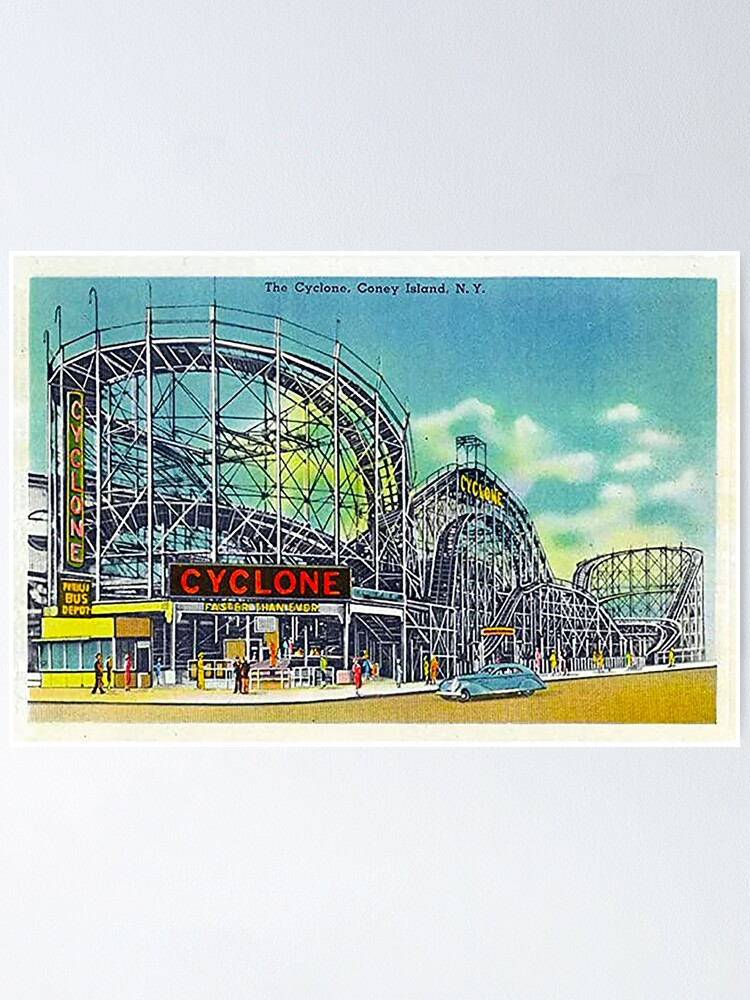The image is of an old cartoonish drawing set within a gray rectangular frame, featuring a postcard-like photograph with a white border. The central focus is the "Cyclone" roller coaster at Coney Island, New York. The roller coaster, depicted in gray and white with visible scaffolding, is prominently labeled "Cyclone" in three places: a black sign with red letters at the bottom front, again in yellow vertical lettering on a building to the left, and within the black-lettered title at the top that reads, "The Cyclone, Coney Island, N.Y." The scene includes a blue sky dotted with clouds, and, below the coaster, an open area resembling an entrance where figures dressed in red, black, and brown stand. Adjacent to the vertical "Cyclone" sign is another that reads "Bus Depot" in yellow on a black background. The road beneath the coaster appears as a brownish-yellow path, and an old-fashioned blue car, likely from the 1940s era, is parked or driving along this road in the center of the image.